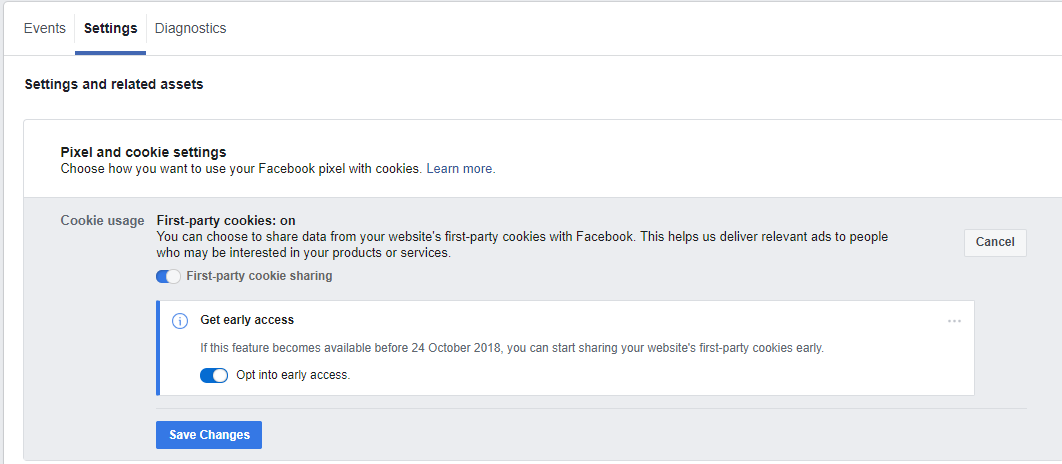The image depicts a section of a settings page on a computer, focusing on Facebook Pixel and cookie settings. At the top of the page, there are three main tabs: "Events," "Settings" (which is more prominently highlighted and underlined with a blue line), and "Diagnostics." Below the "Settings" tab, the page header reads "Settings and Related Assets."

Further down, there is a white rectangular box labeled "Pixel and Cookie Settings." It includes a description: "Choose how you want to use your Facebook Pixel with cookies" and a "Learn More" link. In a section titled "Cookie Usage," there is information about first-party cookies being enabled ("First Party Cookies: On") and an explanation that users can choose to share data from their website's first-party cookies with Facebook to help deliver relevant ads to people who may be interested in their products or services.

This section contains a blue slider labeled "First Party Cookie Sharing," which is turned on. Additionally, there is another white box titled "Get Early Access," which indicates that if this function becomes available before October 24, 2018, users can start sharing their website's first-party cookies early. It includes a slider option ("Opt into Early Access") that is also turned on. At the very bottom of the image, there is a blue button labeled "Save Changes."